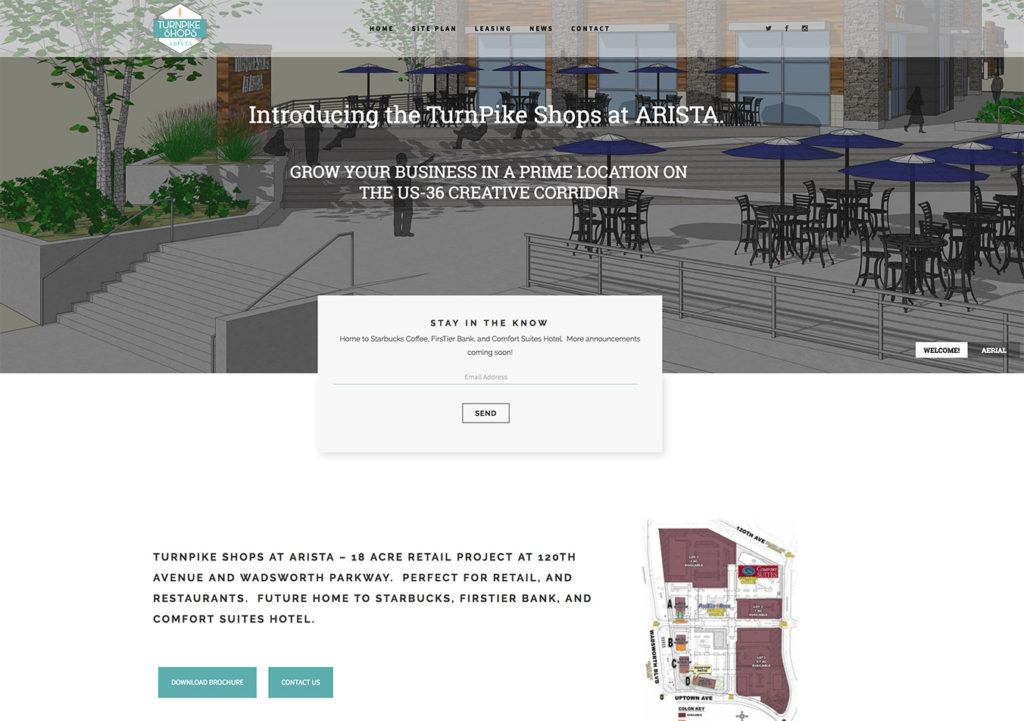The image appears to be a website advertisement for Turnpike Shops at Arista. The upper half of the image showcases a large photograph of a modern commercial building with outdoor seating areas. Rows of tables and chairs with blue and white umbrellas line the front of the building, accompanied by a staircase on the left side. To the right, there is a concrete area with more seating arrangements under matching umbrellas.

At the top of the screen, navigational links are visible, reading: "Home," "Site Plan," "Leasing," "News," and "Contact." The image itself is overlaid with white text that reads, "Introducing the Turnpike Shops at Arista. Grow your business in a prime location on the US 36 Creative Corridor." 

Towards the bottom of the image, a white rectangular pop-up invites visitors to subscribe to updates with the text, "Stay in the know," featuring an input box for an email address and a white "Send" button. 

In the bottom left corner, additional information about the project is presented: "Turnpike Shops at Arista. 18-acre retail project at 120th Avenue and Wadsworth Parkway. Perfect for retail and restaurants. Future home to Starbucks, a first-tier bank, and a Comfort Suites hotel." 

Adjacent to this description, there are two interactive buttons labeled "Download Brochure" and "Contact Us," and to the right, a map is displayed.